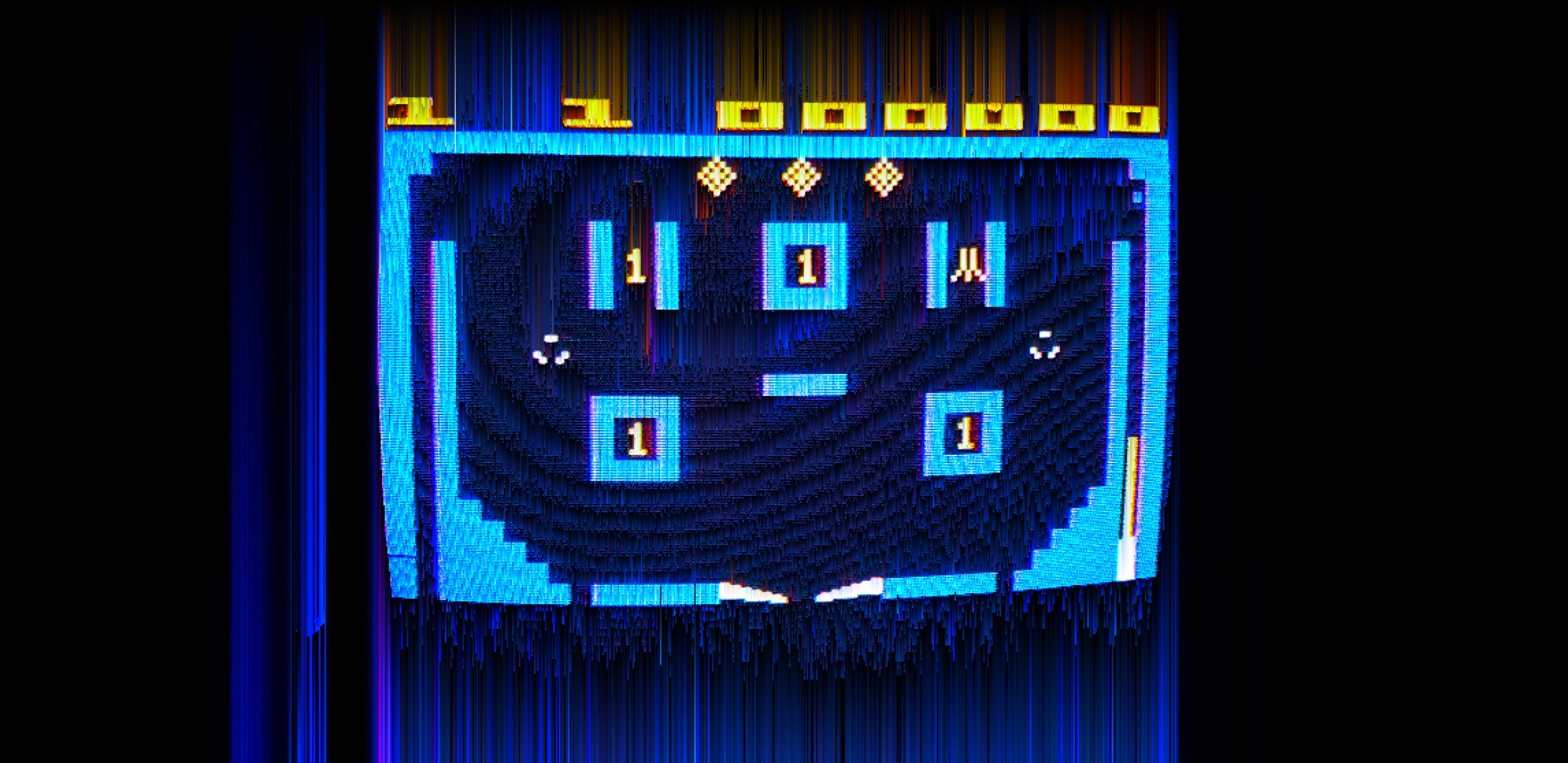This photograph captures an old-school arcade machine featuring a simplistic, retro-style video game. The screen, likely part of a horizontally held gaming device, showcases a dark blue background with lighter blue and aqua elements arranged within it. The main visual includes two prominent white flippers in the middle, resembling a pinball setup. The stage of the game is characterized by blue squares and walls that the pinball bounces off, with each square marked by the number "1". 

There are two parallel blue bars and three squares integrated into the design, along with streaks of blue radiating from the top, bottom, and side, suggesting motion or a graphical effect. The entire display is bordered by a lighter blue frame, enhancing the vintage aesthetic. Dominating the top of the screen are numbers presented in bright yellow: "11" followed by six zeros, possibly indicating a high score or another game-related metric. This nostalgic arcade imagery is set against a black backdrop, giving it a timeless, classic arcade ambiance.